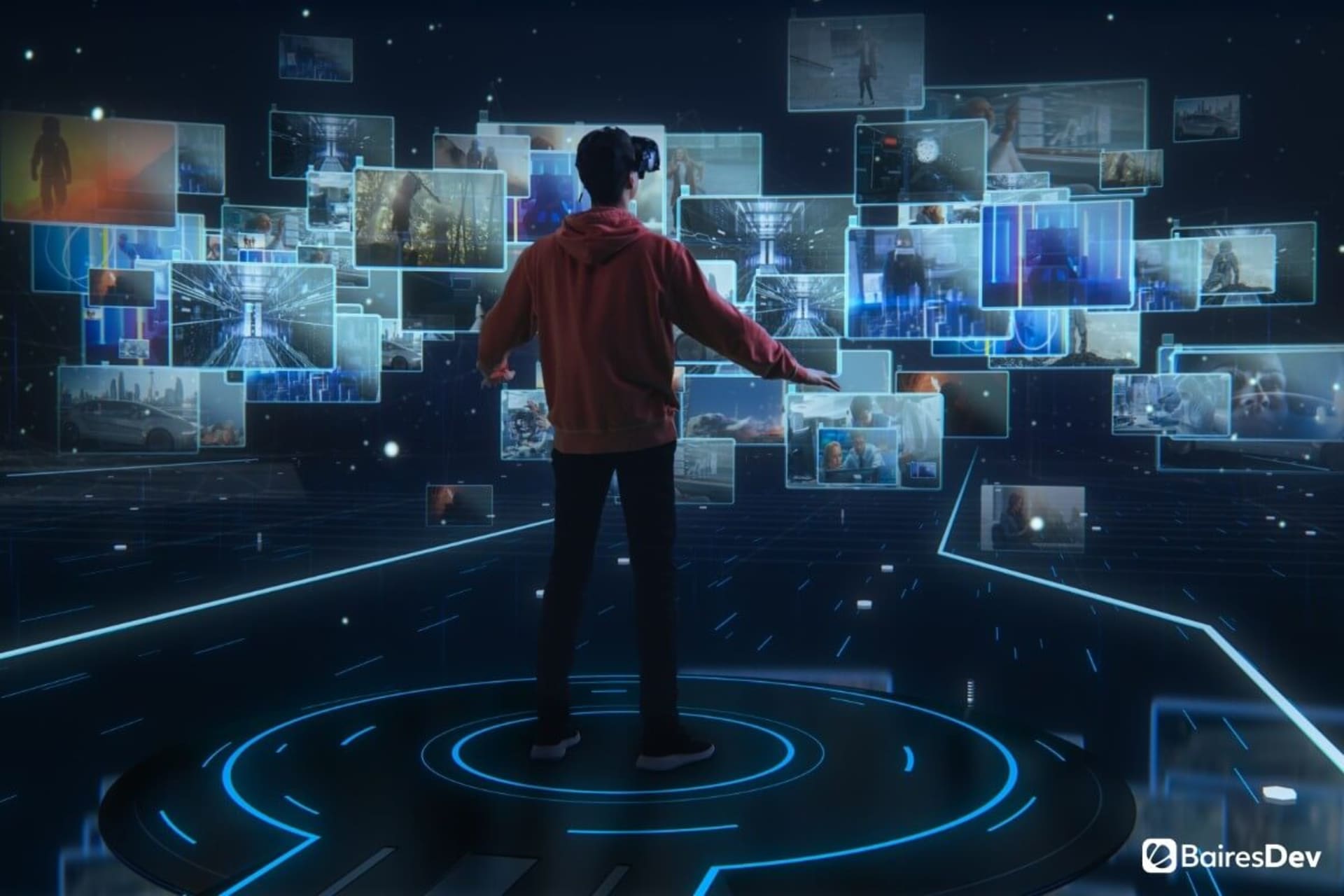In the center of this color image, a man is seen from the back, wearing a dark orange hoodie, jeans, and sneakers. He has his arms extended out to his sides, and he appears to be immersed in a cyber space-like setting. The ground he stands on and the wall behind him are black, interspersed with neon blue and white illuminated lines that resemble the lines between highway lanes, converging into a circle underneath him. The scene has a virtual reality vibe, suggested by the headgear he wears, possibly VR goggles. In front of him, a multitude of digital images projected onto the wall as holograms or suspended screens surrounds him in a curved manner. These screens display various pictures of people, buildings, and hallways, emitting an array of glowing images. The background features a dark sky with small white dots resembling stars. In the bottom right corner, white text reads "BearsDev," likely the name of a company.